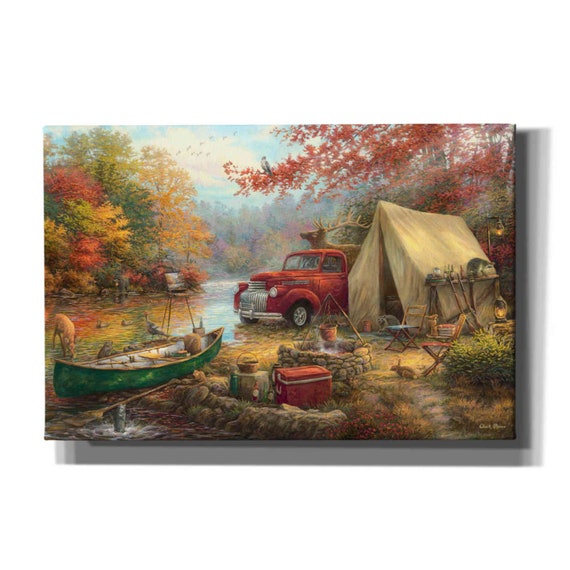The detailed canvas artwork depicts a vibrant camping scene in the midst of autumn. Set against the backdrop of a picturesque woodland with a clear, blue sky and fluffy white clouds, the painting showcases a serene water brook flanked by trees adorned in the vivid hues of fall—ranging from green and gold to burnt orange and brown. To the right, a red, vintage pickup truck is parked next to a pitched tent. Nearby, there are two chairs for campers to sit and enjoy the scenery. On the left, a green canoe is positioned by the riverbank, filled with various camping supplies. Scattered throughout the scene, you can spot a stone fire pit with something cooking, an ice chest, and a couple of seats. The artwork is rich in wildlife, featuring a rabbit, a deer, and a duck amidst the foliage. The overall composition is a colorful tableau of red, yellow, green, and tan tones, expertly capturing the essence of a cozy, autumnal camping experience.